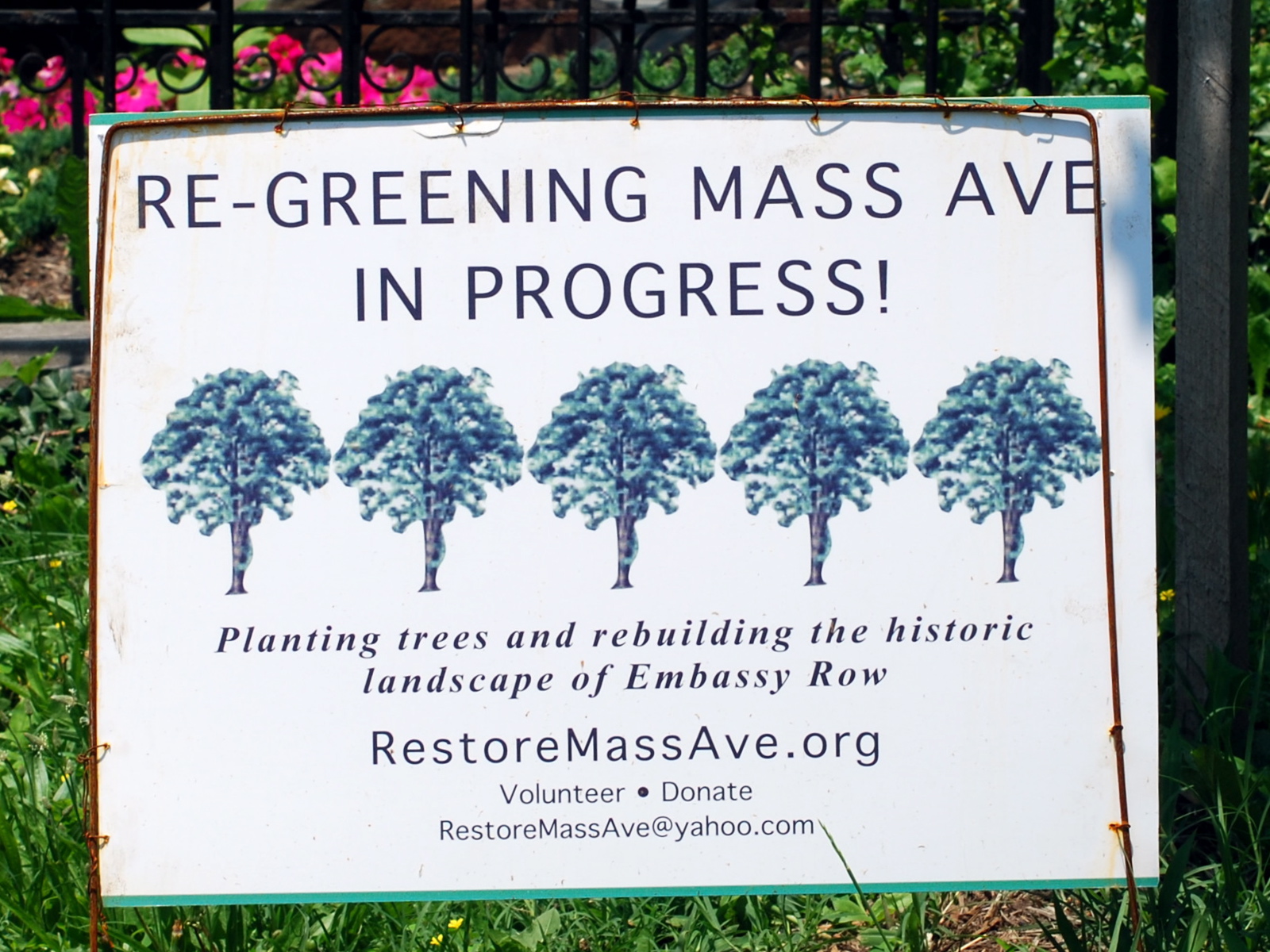The image depicts a weathered sign framed by a slightly rusty metal frame, standing on a green lawn. The sign announces the ongoing initiative to "Re-greening Mass Ave in Progress" with an exclamation mark. Below this headline, the text reads: "Planting trees and rebuilding the historic landscape of Embassy Row." Nested within the sign's central area are images of five identical trees arranged in a row, hinting at the reforestation efforts. 

The lower part of the sign lists "RestoreMassAve.org" followed by prompts for "Volunteer" and "Donate," and ends with "RestoreMassAve at Yahoo.com" in blue text. The sign features thin green stripes along the top and bottom edges and has a predominantly white background. Behind the sign is a wrought iron fence adorned with curling details, partially obscured by green plants and bushes. Pink petunias are visible in the upper left corner above the sign, adding vibrant splashes of color that contrast with the green and white hues. This descriptive sign captures the essence of community efforts to restore and enhance the historic avenue.